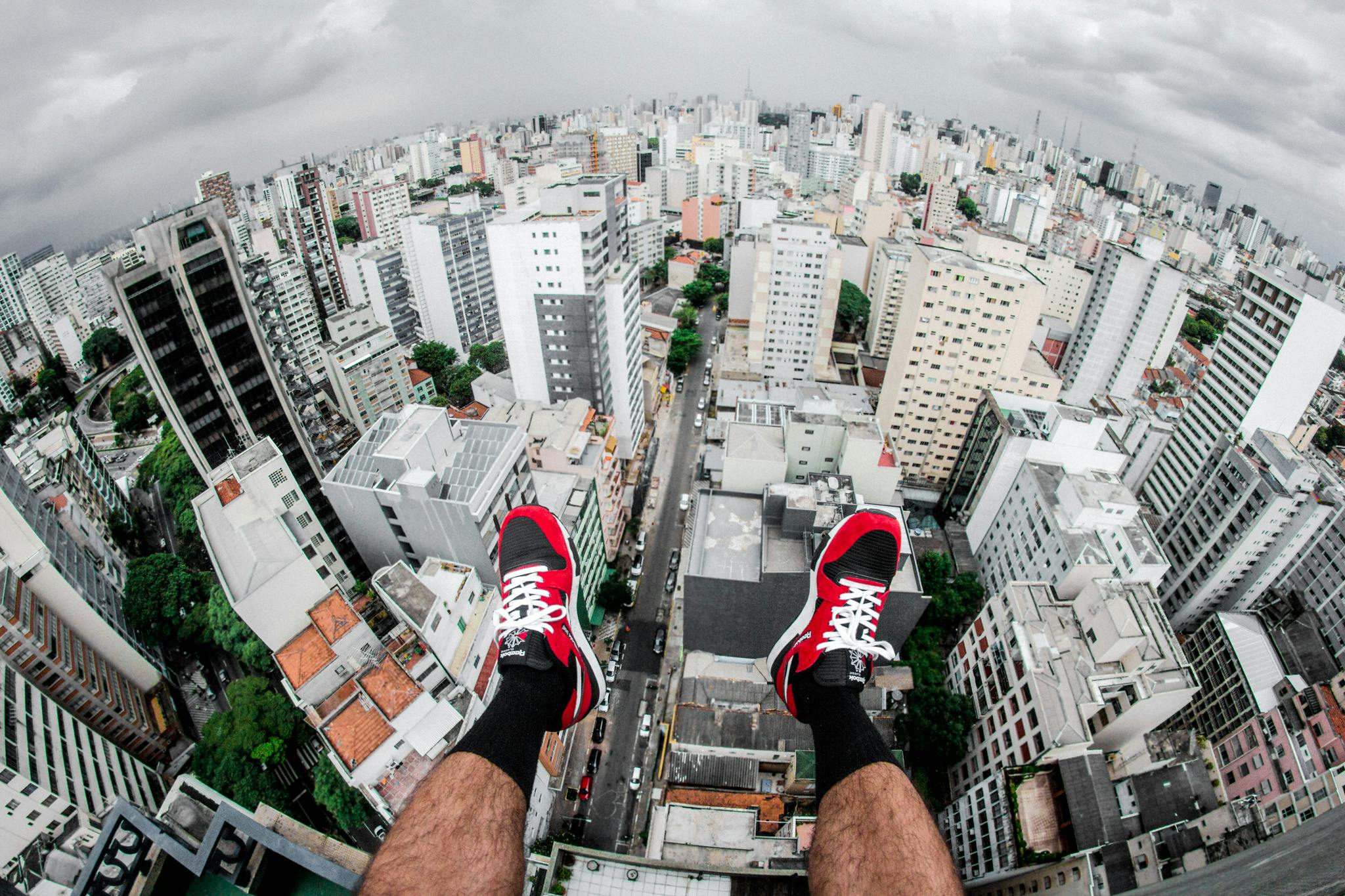In this image, the foreground prominently features a man's lower legs from just below the knees, extending down to his feet. His legs are fairly hairy and of medium complexion. He is wearing black crew socks paired with red and black Reebok running shoes, complete with tied white shoelaces and white soles. The perspective suggests that the photo was taken from a very high vantage point, possibly from a tall building or while parachuting, as his legs dangle over an expansive, densely populated cityscape. The urban landscape below is dominated by numerous tall residential buildings, with a street visible in the scene. The upper part of the image shows a mix of gray and white clouds, reinforcing the high-altitude perspective. Additionally, on the left side of the image, there's a hint of a green park area with visible trees nestled among the buildings, offering a splash of greenery in the concrete jungle. There's no text in the image, leaving the focus entirely on the dramatic overhead view of the city and the man's legs hanging above it.